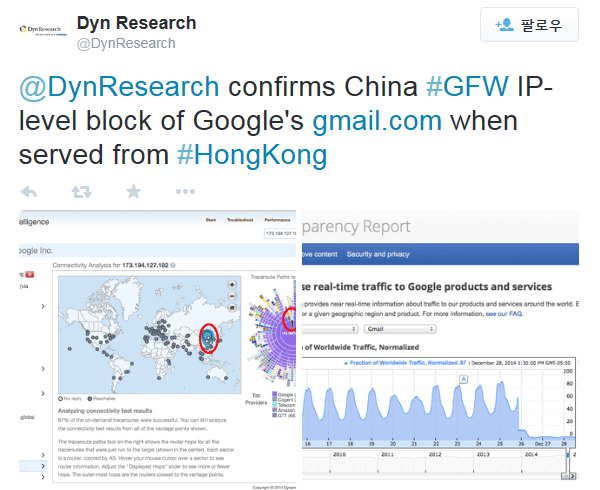**Detailed Caption:**

This image appears to be a social media post from a platform, possibly Twitter, by DIN Research. In the top right corner, there's a symbol featuring a plus icon and a person, alongside Korean characters, indicating it's linked to a Korean service or account.

The post by DIN Research communicates that the organization confirms China's Great Firewall (GFW) is implementing an IP level block on Google's gmail.com when accessed from Hong Kong. Below the text, typical post interaction icons are visible: a left arrow (likely for sharing or replying), a refresh button, a star (possibly for favoriting or bookmarking), and three dots indicating more options.

The image includes two main visual elements:
1. The first visual resembles a Wikipedia-style layout featuring a world map with numerous gray dots. A specific region is highlighted with a red circle showing a blue patch within it, indicating significant data or regions of interest.
2. The second visual element, to the right, features two more data representations. At the top is a circular bar graph also marked with a red circle, labeled "Analyzing connectivity test results," though the detailed text is too small to read. Below this is a graph detailing real-time traffic to Google products and services, showcasing dates ranging from 2010 to 2014 on the x-axis, with numeric data on the y-axis, implying a historical overview of access or connectivity trends.

This detailed data and visual representation aim to portray the impact of China's GFW on Google services, particularly focusing on real-time measurements and historical connectivity trends.